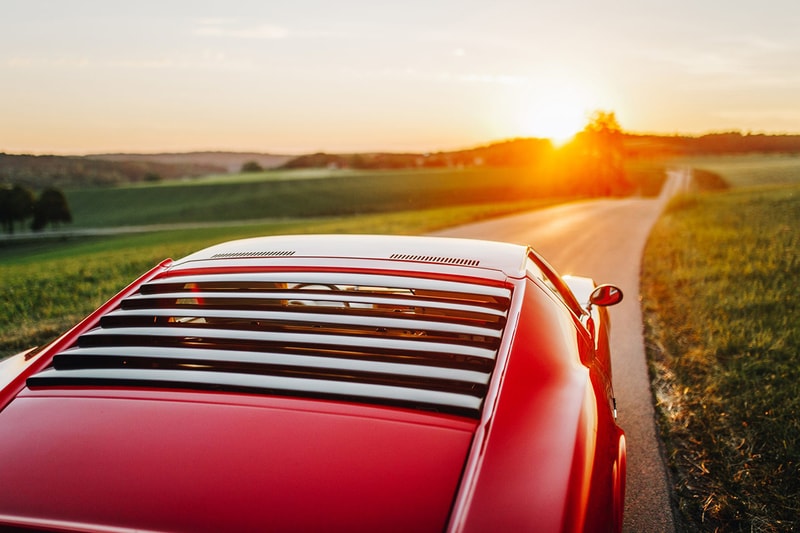The picture features a sleek, modern red sports car, possibly a Mustang, driving on a deserted backcountry road. The road, which has two lanes, extends into a scenic landscape. On either side of the pavement, green grass and rolling hills stretch out, with some trees sprinkled in the far background. The scene is framed by a clear blue sky with the sun setting over distant mountains, creating a picturesque atmosphere. The back window of the car is distinctive, adorned with slats or vents. Tire tracks are visible along the roadside, hinting at previous vehicles that veered into the grass. The predominant colors in the image are the vibrant red of the car, and the natural greens, grays, browns, and whites of the landscape.